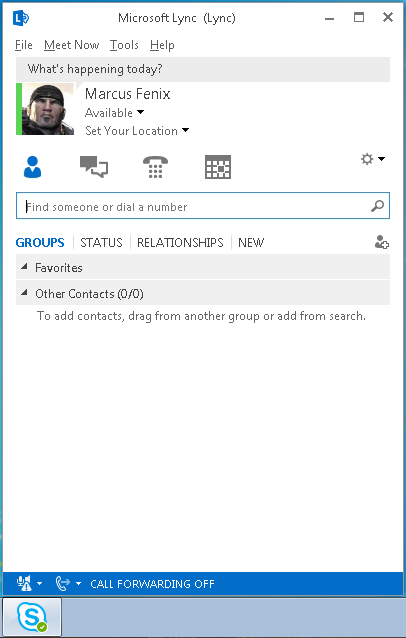The image displays the Microsoft Lync main interface. At the top, the title "Microsoft Lync" is prominently featured alongside the program's icon: a white "L" within a blue square background. Below the title bar, menu options are listed as "File," "Meet Now," "Tools," and "Help."

The central section of the interface displays a header "What's happening today" followed by the user's profile. The user, identified as Marcus Fenix, is shown in a photograph where he is wearing a hat and sporting a slight beard. His eyes are closed, and his expression appears tight. A green border encircles his image, indicating his availability status. There is an option next to his name to set his location.

A toolbar below the header features icons for searching contacts, initiating chats, making phone calls, and accessing calendar functionalities. It includes a person icon with the prompt, "Find someone or dial a number."

Further down, the interface categorizes contacts under sections labeled "Groups," "Status," "Relationships," and "New." The new contacts section has an "Add Person" icon, represented by a person silhouette with a plus sign. In the favorites and other contacts sections, instructions suggest adding contacts by dragging from another group or using the search function. Currently, no contacts are listed for this user.

At the bottom of the interface, it states "Call forwarding off" in white text against a blue background. The very bottom features the Skype logo accompanied by a green check mark, likely indicating the user's connectivity status with Skype.